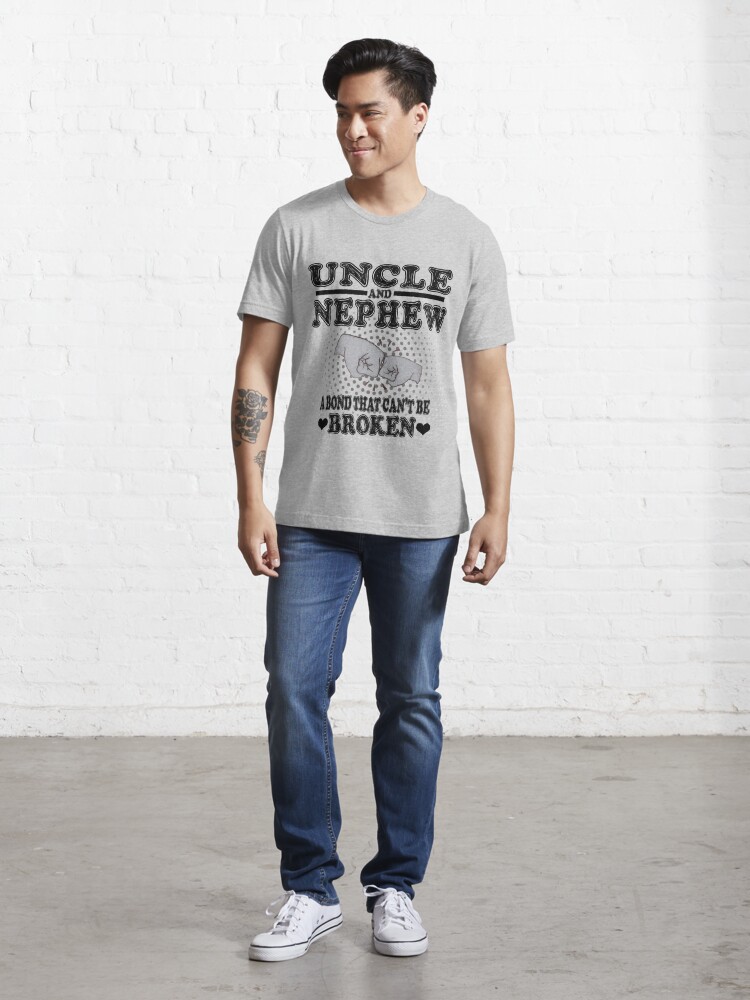The photograph depicts a young Asian man standing on a gray cement floor in front of a white brick wall. His short black hair is styled almost shaved on the sides and longer on top. The man, who is clean-shaven and looking slightly to his right, is wearing white sneakers and blue jeans. His right forearm displays a large tattoo, likely comprised of text that extends along the outside and possibly continues on the inside toward his wrist. He is dressed in a light gray t-shirt featuring black text. At the top of the shirt, it reads "Uncle and Nephew," and below, "A bond that can't be broken," with two black hearts flanking the word "broken." In the center of the text, there is an illustration of two fists bumping each other. The image is full color, vertically rectangular, and appears to have been professionally staged and modeled indoors.